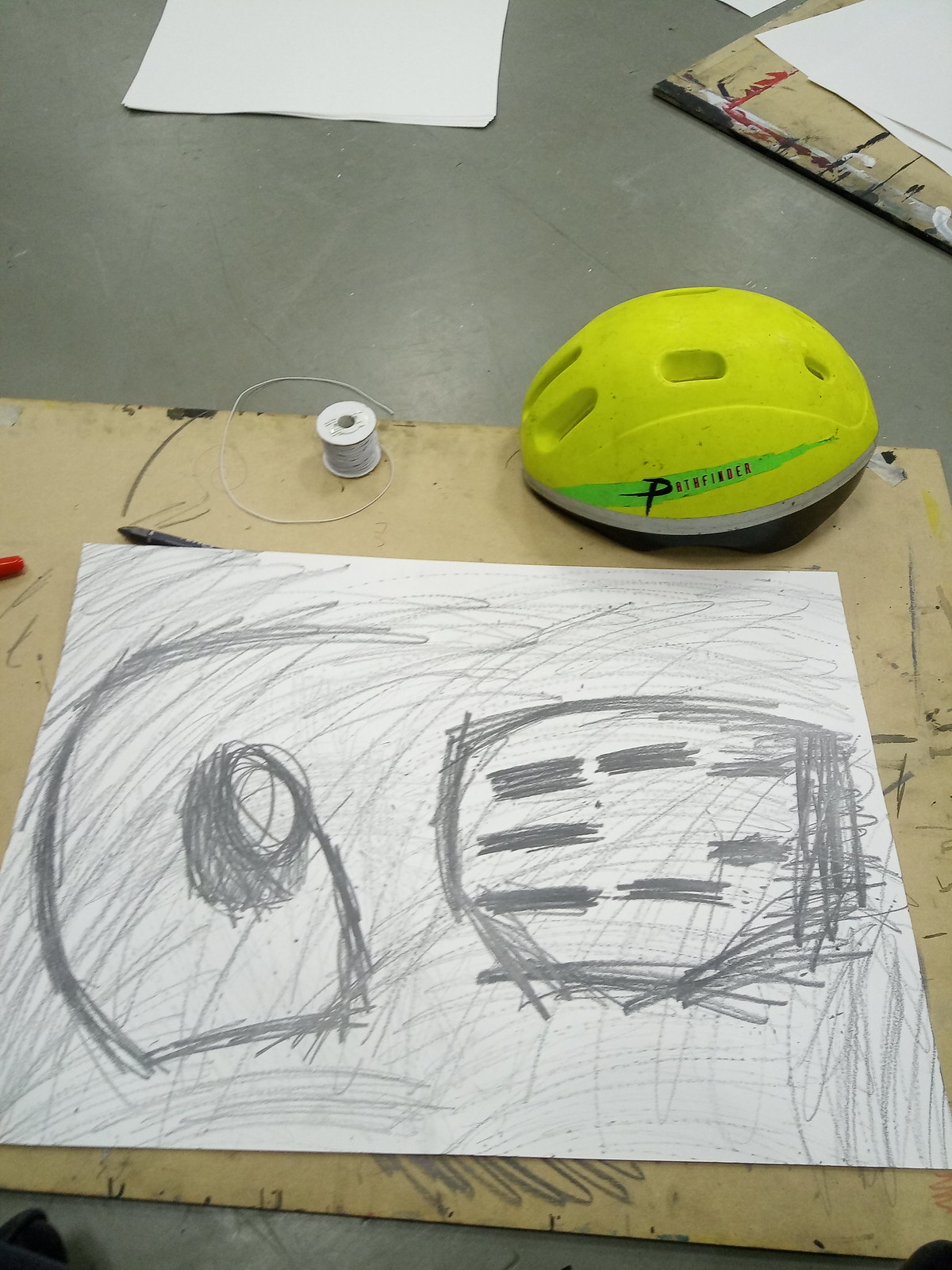This photo showcases an abstract pencil sketch on a white piece of paper, which is placed on a beige cardboard background. The sketch appears to depict various objects with rough, expressive lines and shapes. Dominating the sketch is a central circular shape with a smaller clear circle inside it, accompanied by a curling line that extends out and curves down and up, resembling an eyeball or spool of thread. On the right side of the sketch, there is an almost box-like figure filled with multiple thick horizontal lines, likely representing an object with a textured surface.

Surrounding the sketch are several notable items. In the background to the right, there is a yellow and green child's bike helmet that features a green arrow-shaped line and is accented with gold trim and a black base. The helmet has the brand name starting with the letter 'P' in black lettering. To the left of the drawing, there's a white spool of thread with stray threads extending away from it. Additionally, there's a black pen partially visible behind the white paper, a red pen tip, and another beige cardboard piece displaying splashes of red, white, and black paint. Scattered above the main drawing are several sheets of blank white paper on what appears to be a gray desk or table, enhancing the creative and somewhat cluttered setting of the scene.